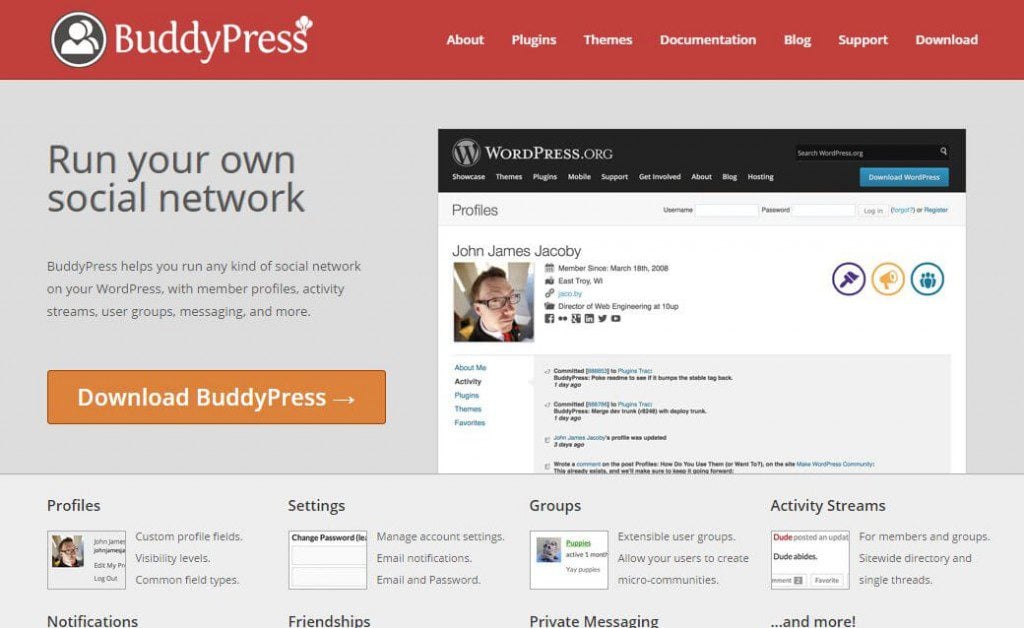The BuddyPress website features a prominent design that clearly showcases its purpose and functionalities. At the top of the page, a long red bar spans across the screen, prominently displaying the site name "BuddyPress" in white text on the left side. Situated just above the last 'S' of 'BuddyPress' are three small, white balloon icons. To the left of the site name is a circular icon depicting two people, also in white.

Navigationally, the top bar includes seven categories for users to explore: About, Plugins, Themes, Documentation, Blog, Support, and Download.

The middle section of the screen prominently highlights BuddyPress's key message: "Run Your Own Social Network." Directly beneath this message, a detailed description states: "BuddyPress helps you run any kind of social network on your WordPress with member profiles, activity streams, user groups, messaging, and more." An eye-catching, large orange rectangular button labeled "Download BuddyPress" with a right-pointing arrow encourages immediate action.

On the right half of the middle section, there's an inset black bar at the top with "WordPress.org" displayed in white text on the top-left corner. Below this, various icons are lined up horizontally. Further down, a profile section showcases John James Jacoby—visually represented as a man wearing glasses and a suit, with white objects in the background. Some additional information appears to the right, though it's not fully legible.

Directly beneath this profile section, a gray inset box presents a bullet-point list, although the details are unclear.

Occupying the bottom third of the page, a long gray bar introduces four main categories:
1. **Profiles**: Featuring a small screenshot of John James Jacoby's profile with a brief description to the right mentioning "custom profile fields" and additional features.
2. **Settings**: Illustrated with an image suggesting options to "change settings" and "change passwords," accompanied by descriptive text.
3. **Groups**: Although the accompanying image is not clear, the description to the right mentions "extensible user groups."
4. **Activity Streams**: Paired with an image, featuring notes about a "statewide directory" and "single threads."

Towards the bottom of this gray bar, four more categories are listed: Notifications, Friendships, Private Messaging, and More. These categories are intended to highlight additional functionalities of BuddyPress.